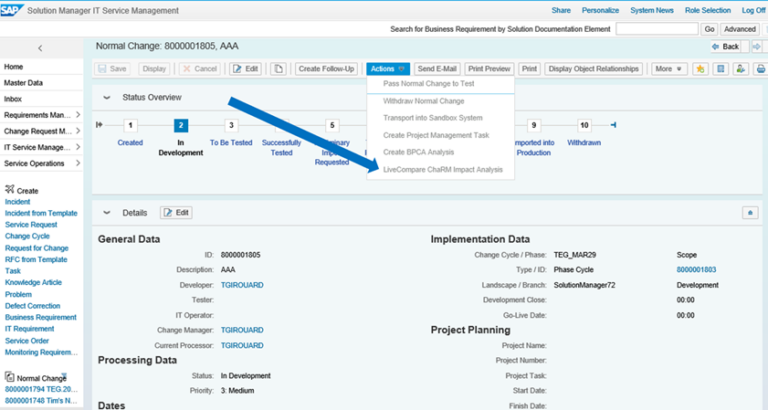The image depicts a computer screen displaying a webpage for SAP Solution Manager IT Service Management. At the top, the page header has 'SAP' prominently displayed in white capital letters within a blue tab. Below this header, the main section of the page features a faint blue background.

To the left of the screen, there is a vertical menu with various clickable options listed in black text. These menu options include:
- Home
- Master Data
- Inbox
- Requirements
- Man...
- Change
- Request M.
- IT Service Manager
- Service Operations

To the right of the left-hand menu, there is a segment labeled 'Create' which includes a list of blue hyperlinks. These links are:
- Incident
- Incident from Template
- Service Request
- Change Cycle
- Request for Change

Additionally, a blue arrow digitally overlays the screen, directing the viewer's attention towards the right and downward. This arrow points to a specific part of the screen featuring a drop-down menu that includes the options:
- Live
- Compare
- CHAR or CH
- RM Impact Analysis